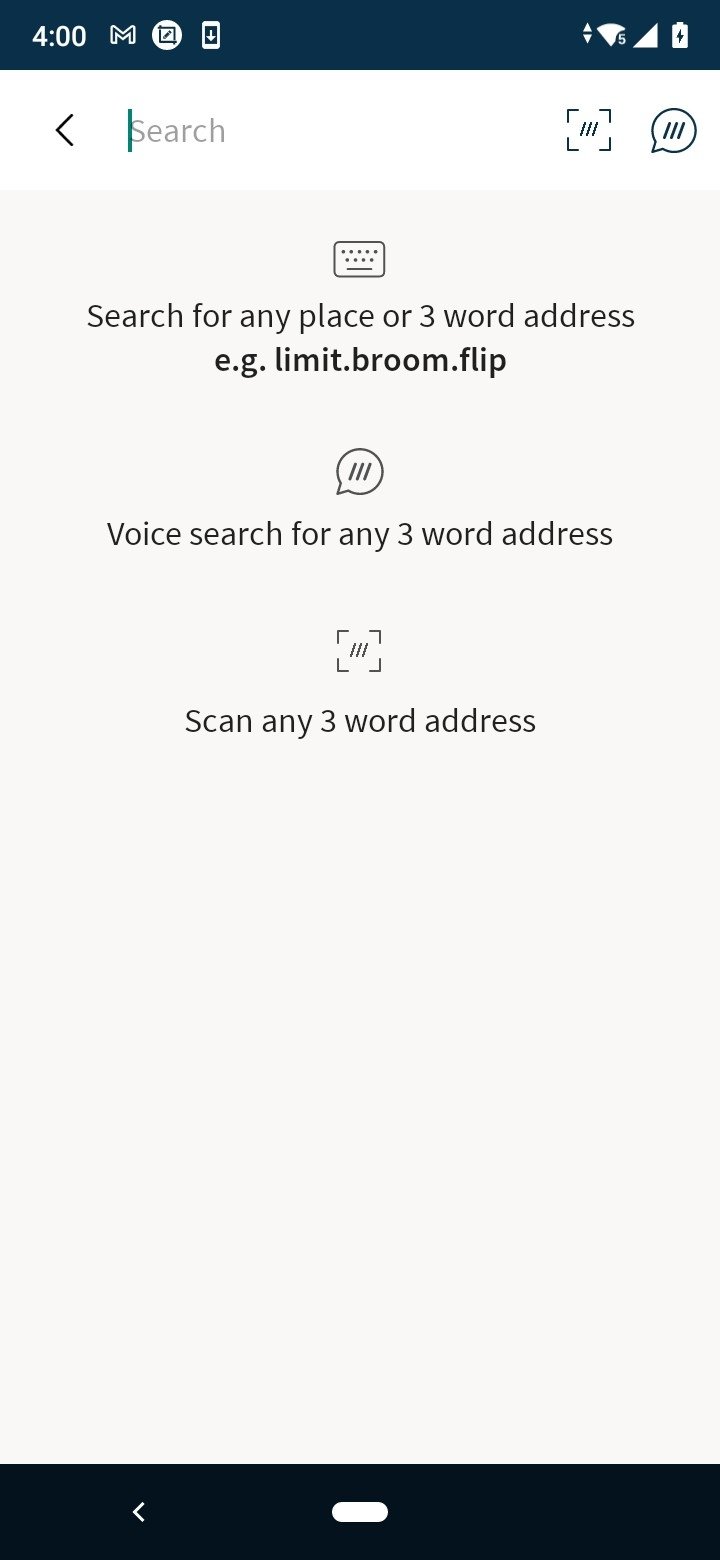A detailed image caption would be:

"The image displays a smartphone screen with a user interface for search navigation. At the top of the screen is a dark banner, either navy blue or black, displaying the time (4:00 PM) on the far left, followed by a mail icon (M), and a couple of additional icons. To the far right of this banner, the icon shows a fully charged battery with all five bars. Below this, a white banner spans the screen's width; on the left side of this banner is a black back arrow. Next to the arrow is a search bar with the word 'Search' faintly displayed in light gray, and a bright blue cursor positioned just before the 'S'. The right side of the banner features a text icon and another unidentified icon. The main background color of the screen below this white banner is light gray. At the top of this section in gray text is the prompt 'Search for any place or three-word address.' Below this prompt, in bold black text, is the example address 'E.G.Limit.Broom.Flip.' Further down, a text icon is visible with a subsequent gray text instruction, 'Voice search for any three-word address,' followed by another gray instruction, 'Scan any three-word address.' At the very bottom of the screen, a black ribbon stretches across the width."